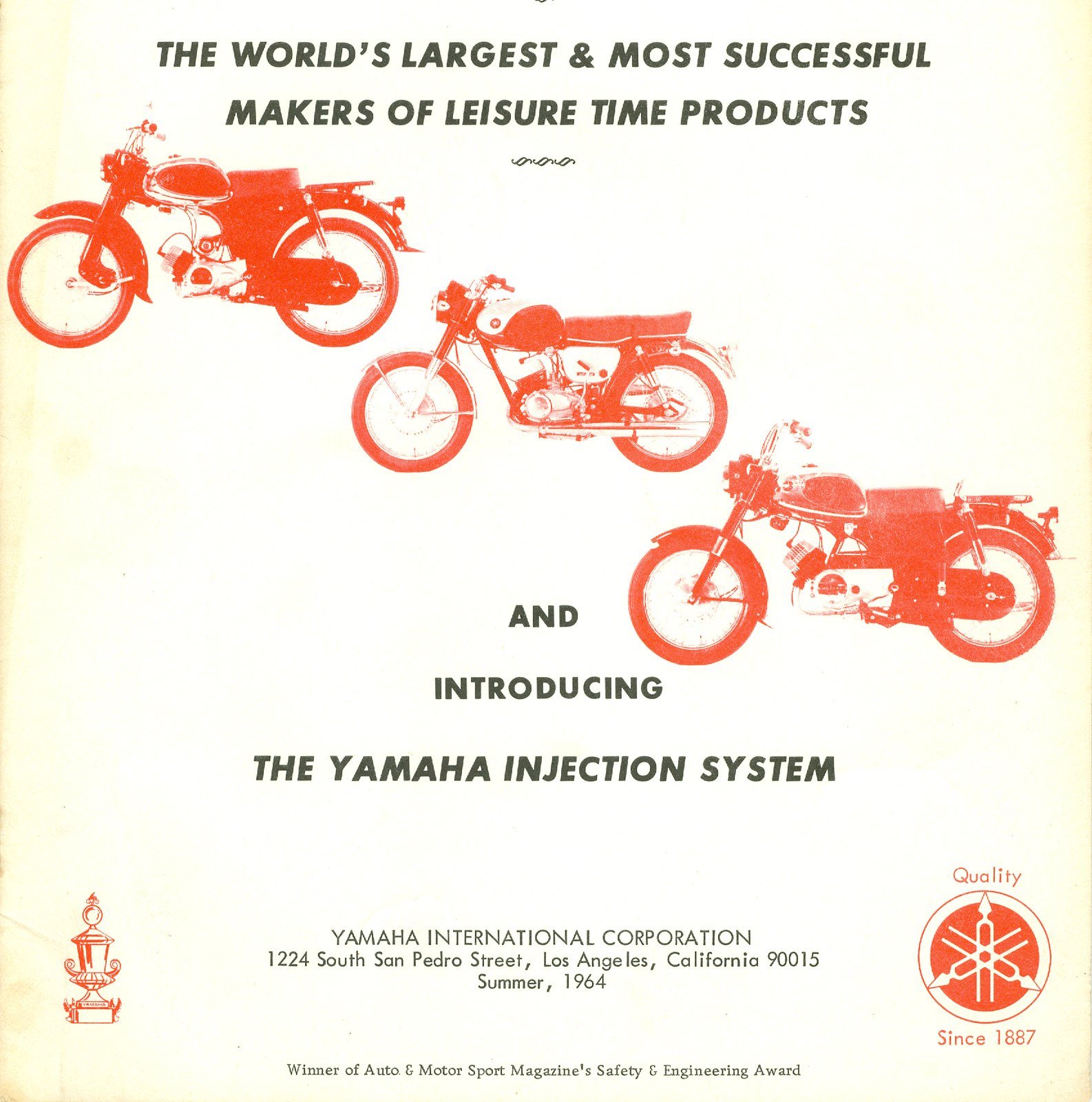The advertisement features a wide vertical rectangular shape with a light beige background. At the top, centered in black text, it reads, "The world's largest and most successful makers of leisure time products." Diagonally from left to right, three red sketch drawings of different Yamaha motorcycles are prominently displayed. Below the motorcycles, centered in black, are the words, "And introducing the Yamaha Injection System." Further down, also centered, it says, "Yamaha International Corporation," followed by the address, "1224 South San Pedro Street, Los Angeles, California, 90015." The caption notes "Summer 1964" beneath the address and at the very bottom, in very small print, it reads, "Winner of Auto and Motorsport Magazine Safety and Engineering Award." Additionally, on the left side of the advertisement is a small red trophy illustration, and on the right, a circle bearing a logo with the text, "Quality Since 1887."